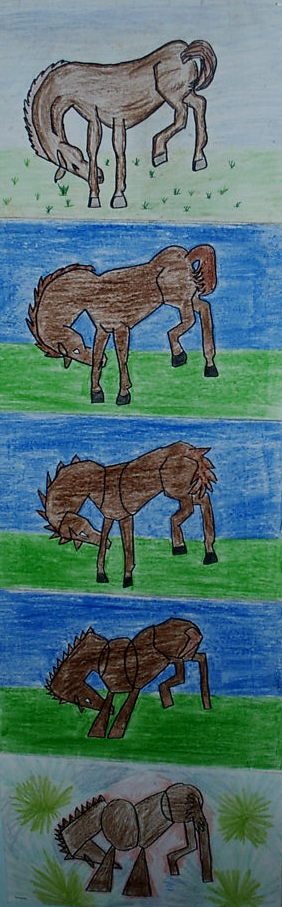The image is a tall, narrow strip consisting of five progressively detailed drawings of a horse, which seem to serve as a step-by-step guide on how to draw one. Each horse is depicted standing diagonally, with its hindquarters towards the top right and its head lowered towards the bottom left, as if grazing. They are colored predominantly in shades of brown with green grass beneath their hooves and a blue sky in the background, except for the initial drawing which only includes the grass. The progression begins at the bottom with a basic sketch formed by circles and triangles, moving upwards, each drawing becoming more refined. The topmost drawing showcases a detailed rendition of a horse with varied shading, using crayons or colored pencils to achieve a more lifelike appearance. Notably, the middle drawings distinctly feature black hooves, while some of the earlier illustrations omit this detail. Each horse is set in what appears to be a field, indicated by the grassy and open blue sky setting.